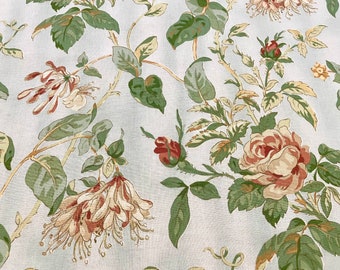A photograph of a white cloth, possibly a tablecloth or curtain, intricately decorated with a vibrant array of flora. Dominating the right side is a large, fully bloomed flower with striking red and white petals, serving as the centerpiece. Surrounding this main flower, there are several other floral elements: on the upper portions, green leaves and vines feature prominently, accompanied by white bulbs tinged with red interiors that have yet to blossom. Adjacent to these, a red flower still in its bud stage can be observed. Additionally, pink roses in various stages of blooming appear throughout the fabric, with a particularly distinct pink flower in the bottom right. A few yellow flowers add diversity to the color palette, and some leaves even exhibit a subtle gold tint. This floral design creates an enchanting and lively aesthetic, ideal for springtime gatherings such as tea parties or festive dinners.